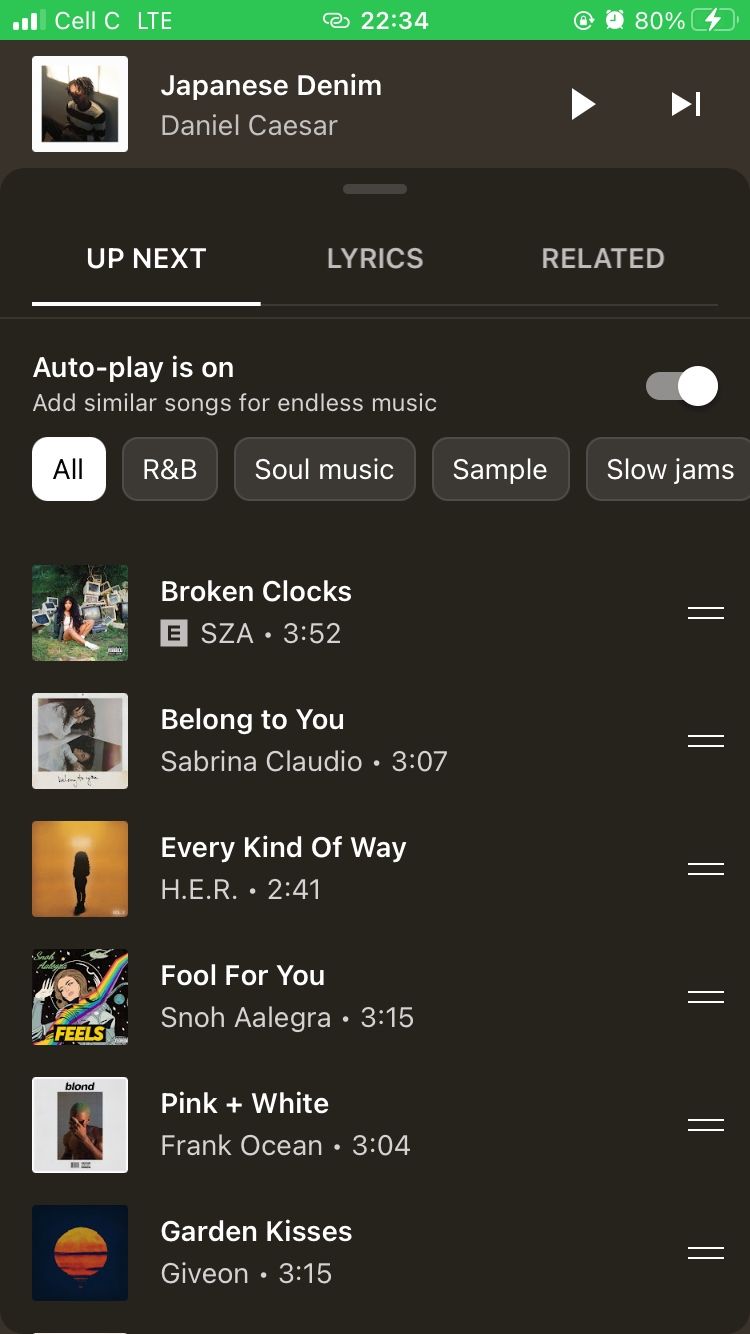### Descriptive Caption

A smartphone screen displaying a music app interface is seen. The top part of the screen features a green status bar that shows various indicators: on the left are the signal strength bars, in the center it reads "LTE" indicating the data connection type, and to the right it displays the time "22:34." Next to the time, there are icons for a lock, an alarm, and an 80% battery indicator.

Beneath the status bar, the screen has a predominantly black background with text and icons. The large text reads "Japanese Denim" indicating the current song title. Below this, the name "Daniel Caesar" is displayed, along with a right-facing arrow and an arrow with a line through it, likely indicating navigation options. The central part of the screen features a thumbnail image of a smiling black man with ear-length curly hair, wearing a red and white striped t-shirt and blue jeans.

Further down, informational text says "Up Next," followed by "Lyrics and Related." It then specifies that "Auto Play" is on and that similar songs will be added for continuous music playback.

The bottom section of the screen lists the next six songs in the queue, each accompanied by a small image:
1. "Broken Clocks" by SZA, duration 3 minutes and 52 seconds.
2. "Belong to You" by Sabrina Claudio, duration 3 minutes and 7 seconds.
3. "Every Kind of Way" by H.E.R., duration 2 minutes and 41 seconds.
4. "Fool for You" by Snoh Aalegra, which is partially visible. 

The music genre prominently featured is R&B/Soul, focusing on slow jams.